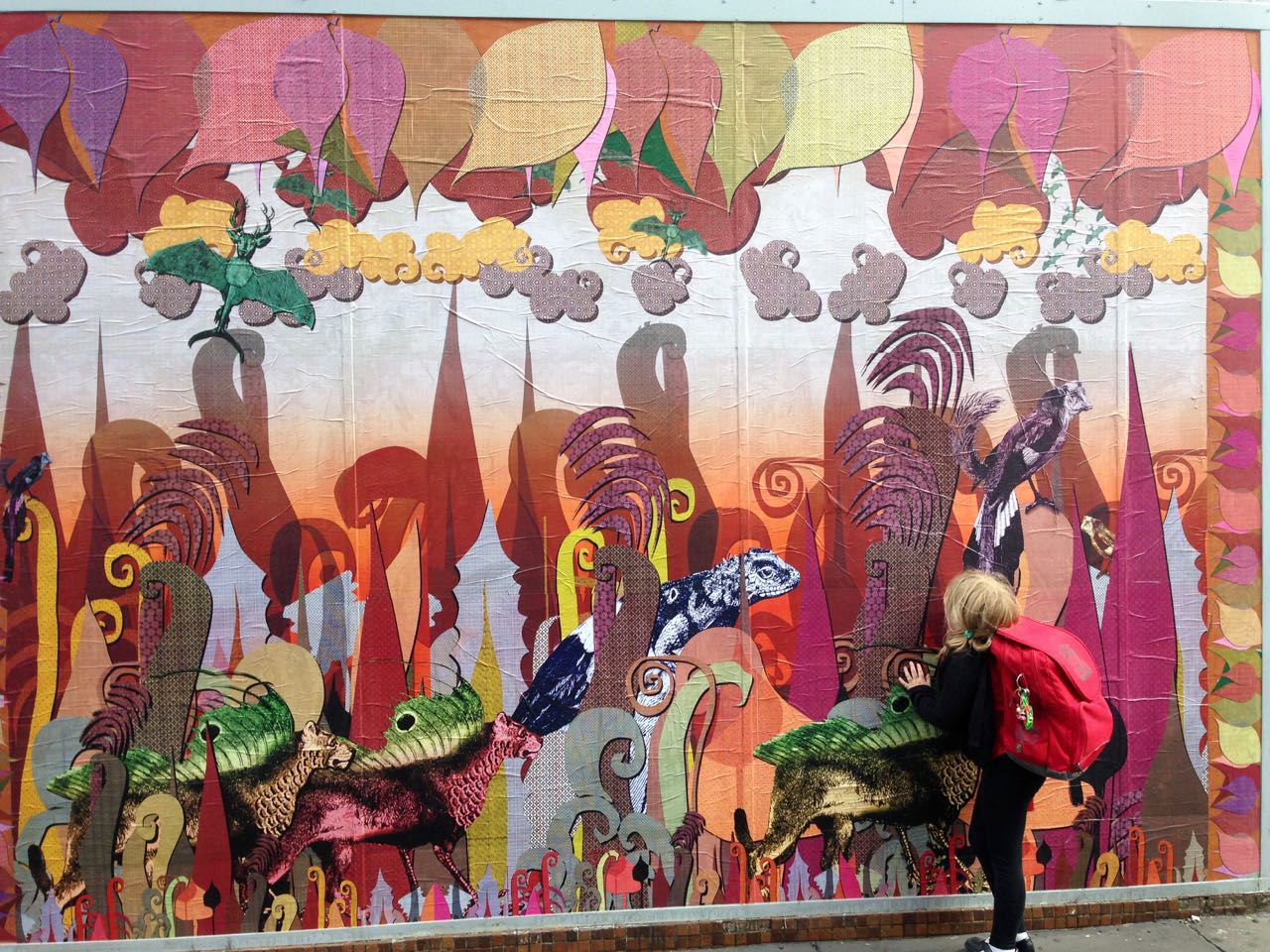A vibrant and whimsical mural adorns a city wall, bursting with bright hues of purple, red, pink, yellow, and orange, especially prominent in the balloon-like drawings across its top section. Below these, puffy clouds in shades of gray and yellow float above a fantastical blend of a forest and a Gothic-style cityscape, teeming with various painted animals such as tortoises, cheetahs or hyenas, iguanas, parrots, and peculiar caterpillar-like creatures. Strange, illustrated trees and plants add to the mural's enchanting atmosphere. In the foreground, standing on a gray concrete sidewalk in front of a reddish-brown brick portion of the wall, is a child, approximately 10 years old with short blonde hair, dressed in a long-sleeved black shirt, black leggings, and tennis shoes. The child, with their face close to the mural and their back to the camera, wears a large red backpack adorned with keychains, captivated by the vivid scene before them.